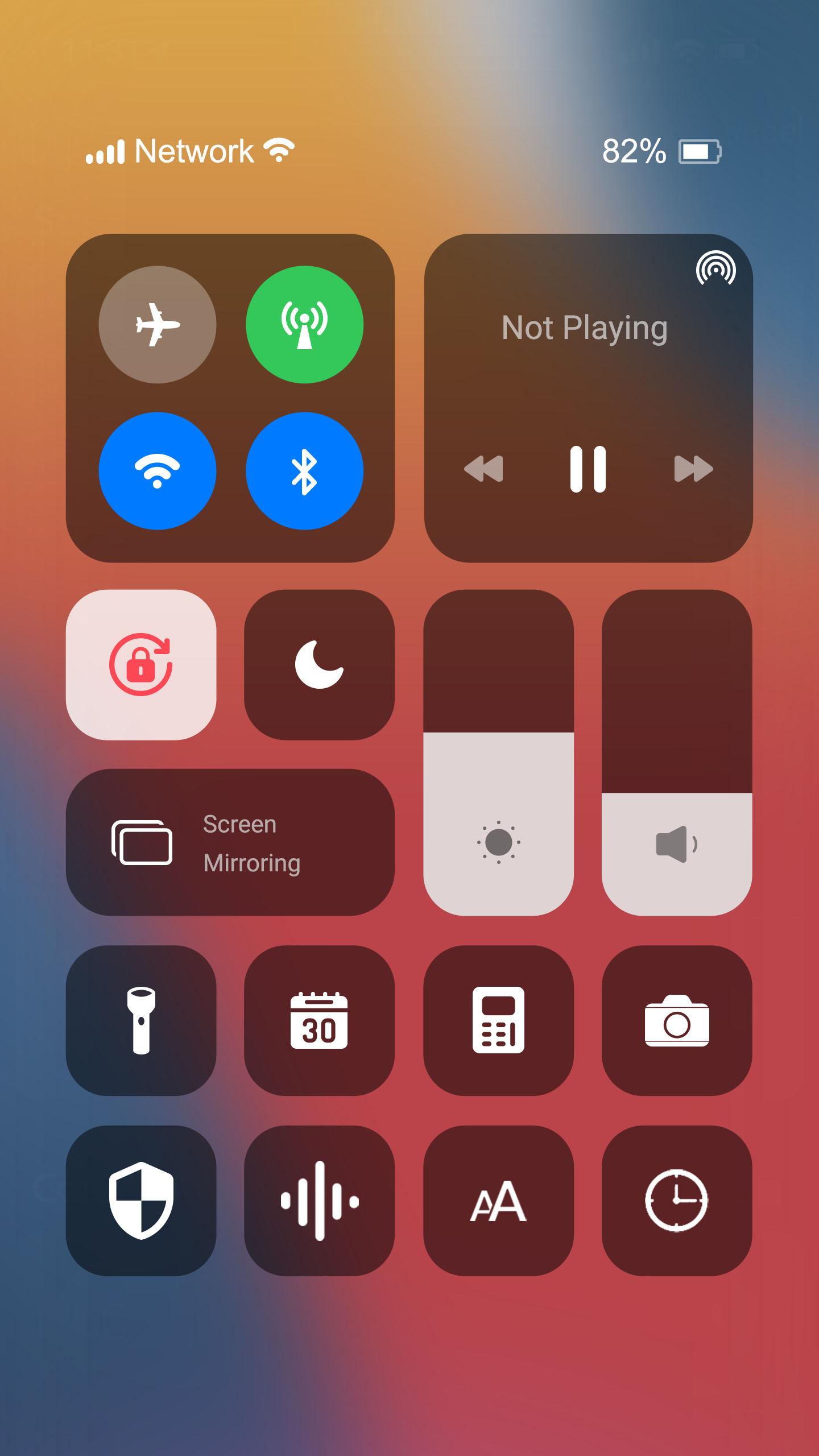This image showcases a detailed view of a smartphone's control center interface. At the top left corner, there's a "Network" label accompanied by a Wi-Fi icon, and directly to the right is an "82% battery life" indicator. 

Below, there's a black square featuring several connectivity icons including Wi-Fi, Bluetooth, cellular data, and an inactive airplane mode. Adjacent to this square is a "Not Playing" placeholder, suggesting that no media is currently being played. 

Further down, a row of icons is arranged: a screen rotation lock, a "Do Not Disturb" icon, a "Screen Mirroring" option, a brightness slider, and a sound level control. 

Beneath these elements are eight squares representing various utilities: a flashlight, a calendar (labeled as "Day"), a calculator, and a camera. Below these are a shield icon, a data usage icon, a text icon, and a clock icon. 

The background gradient features multiple colors: blue in the bottom left and top right corners, a predominant pink hue spanning the majority of the interface, and a yellow-orange tint in the top left corner. This colorful background seamlessly integrates with the control center elements, creating a visually appealing interface.